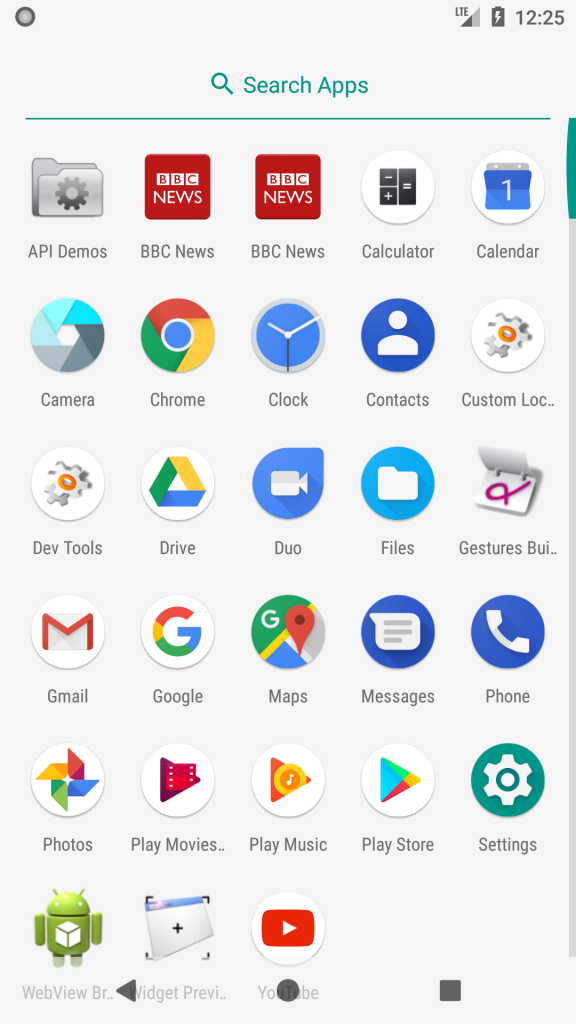The image depicts a section of a digital interface set against a light blue background predominantly in the upper left corner. In this portion, there is a black circle with the time displayed as 12:25. Adjacent to it, in green text, is the phrase "Search apps," accompanied by a small magnifying glass icon. Below this, a green line separates this section from the array of icons below.

The main area features a comprehensive grid of application icons, including: API Demos, BBC News (listed twice), Calculator, Calendar, Camera, Chrome, Clock, Contacts, Custom Location, Developmental Tools, Drive, Duo, Files, Gestures, Building, Gmail, Google, Maps, Messages, Phone, Photos, Play Movies, Play Music, Play Store, Settings, Web View Browser, Widget Preview, and YouTube.

At the bottom of the interface, there are three navigational icons in gray— a triangle, a circle, and a square—presumably representing the standard back, home, and recent apps buttons. At the very bottom, the image displays the "Web View" label, highlighted by a green slider button on the right-hand side.